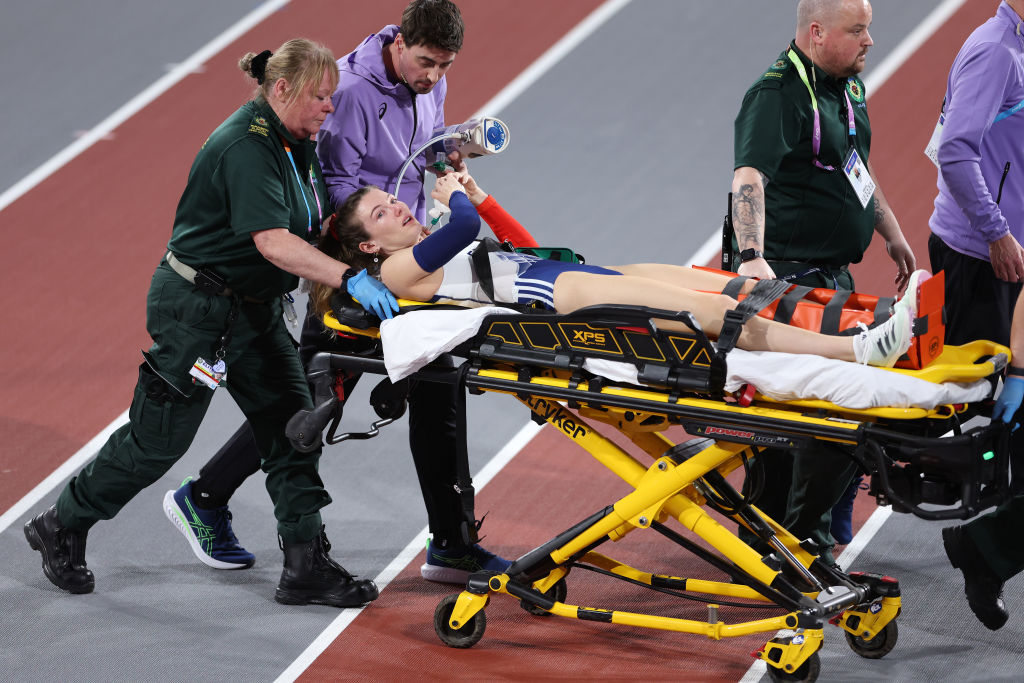In this high-resolution photograph, a young female track and field athlete, who appears to be in her early 20s, is being taken off the track on a yellow and black stretcher after sustaining an injury. She has an orange splint securing her left leg extending past her knee. The athlete, who is white, wears a white track suit comprising a white tank top and short blue running shorts with three white stripes on the side. Additionally, she sports white running shoes featuring three green stripes. The expression on her face reflects concern as she looks directly at the camera, holding an item near her head. 

Medical personnel, dressed in distinctive uniforms, are actively assisting in her transport. The scene includes a woman in compact green fatigues pushing the stretcher, another staff member in purple attire handling a medical device, and two other individuals—possibly from security—walking ahead. There are also three people in front of the stretcher with their hands on it, coordinating its movement. The team's coordinated effort underscores the urgency of the situation, highlighting the severity of the athlete's injury.